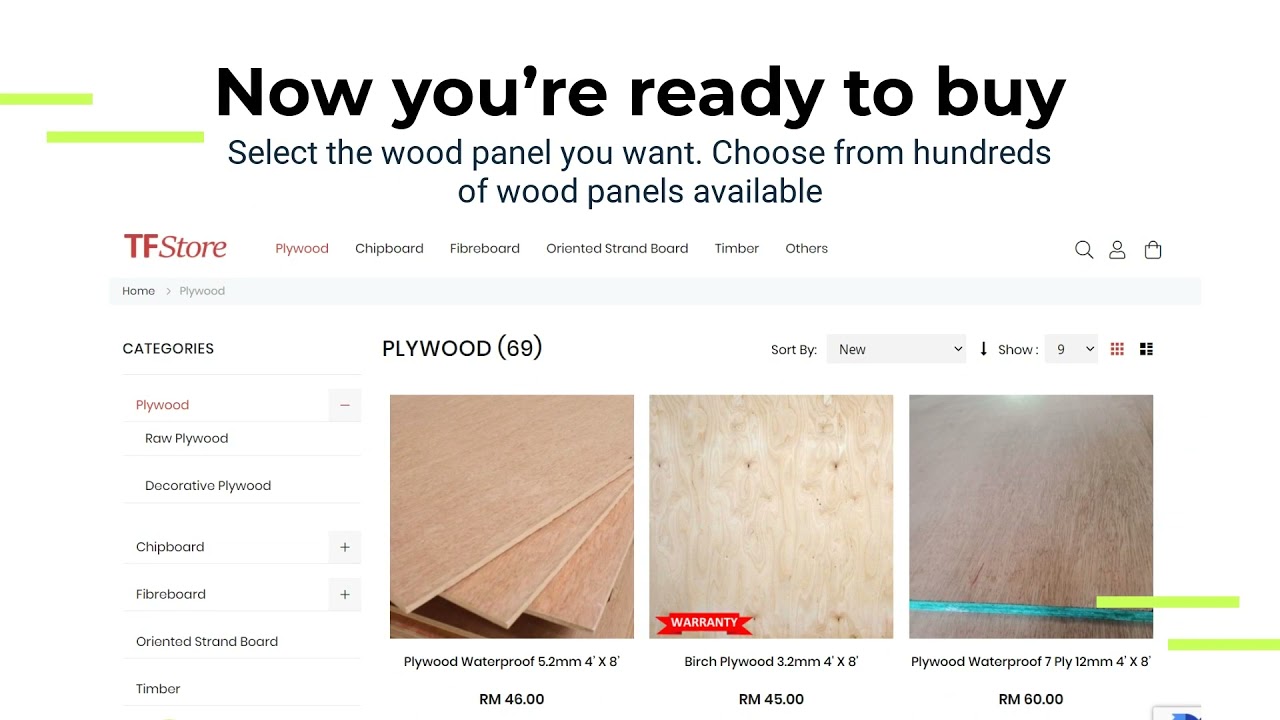Caption: 

A user interface for the TF Store website showcases a sleek, white background with vibrant red accents. At the top left, the store’s name, "TF Store," is prominently displayed in bold red letters. The interface invites customers to select from a diverse array of wood panels, with a call-to-action prompt reading, "Now you're ready to buy. Select the wood panel you want, choose from hundreds available." 

Below this prompt, the categories are clearly organized. Each category title is listed in black, but "Plywood" stands out in eye-catching red. The plywood category itself is further divided into subcategories, including waterproof plywood, birch plywood, and more specialized types such as decorative plywood, chipboard, fiberboard, oriented strand board, and timber. Each subcategory lists detailed information about the available products, including the type, measurements, and prices. 

For instance, the first product highlighted is waterproof plywood measuring 5.2 millimeters and sized at 4 by 8 feet, priced at $46. Following this is birch plywood, also 4 by 8 feet, marked at $45. Another type of waterproof plywood, again 4 by 8 feet, is displayed with a price tag of $60.

On the right-hand side of the interface, functional icons for search, user account, and shopping cart streamline the user experience. The categories section reinforces the selection with a concise list and an ability to sort products by new arrivals and display options, such as showing nine items per page.

In summary, the user interface of the TF Store is straightforward, user-friendly, and richly detailed, making it easy for customers to navigate and choose the wood panels suited to their needs.